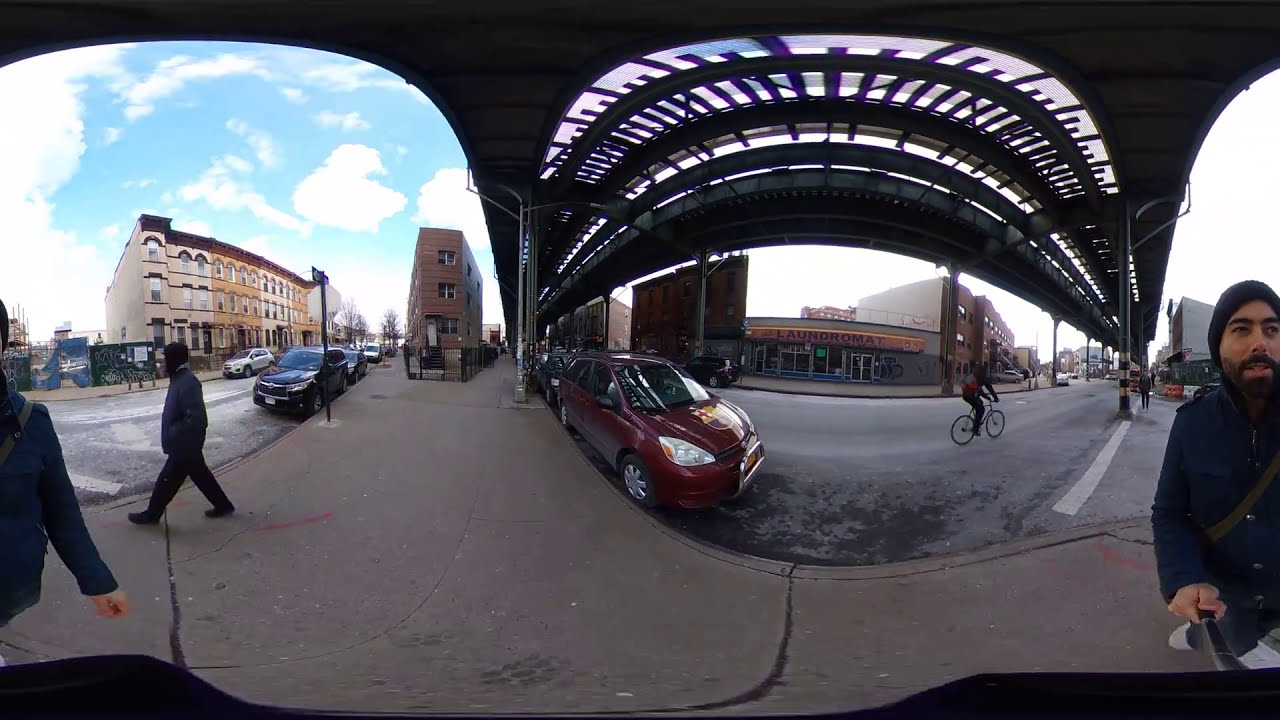This outdoor daytime photograph captures an urban cityscape viewed from beneath a prominent black metal arched structure, likely part of an overhead railway or travel station. The arch, characterized by its looping design, frames a blue sky with puffy white clouds. Below the arch, an urban street stretches out, flanked by buildings of varying heights and architectural styles. 

On the left side of the image, a large light-colored building with a dark brown or red roof stands three to four stories high, potentially serving as a hotel, office building, or apartment complex. To its right, a narrower, three-story dark red brick building with a flat roof is noticeable. Between these two structures, a street extends down the middle, populated with parked cars and pedestrians.

People are actively moving along the sidewalk adjacent to the narrow building, which is described as having a "dirty" brown cement surface. Among the visible pedestrians is a man in the foreground wearing a dark hat, sporting a mustache and beard, and donned in a blue jacket. His right arm extends out, holding an unclear object that could be a bicycle or luggage handle.

The street curves in a U-shape toward the viewer's perspective, creating a dynamic flow in the scene. Near the bend of the road, a red car is parked facing right, while a bicyclist is seen heading towards the background. On the right side of the image, the landscape features additional urban buildings, including one that likely houses a laundromat, adding to the bustling city ambiance.

This image encapsulates an everyday urban moment, blending the structural elements of the railway arch with the lively street scene beneath it.